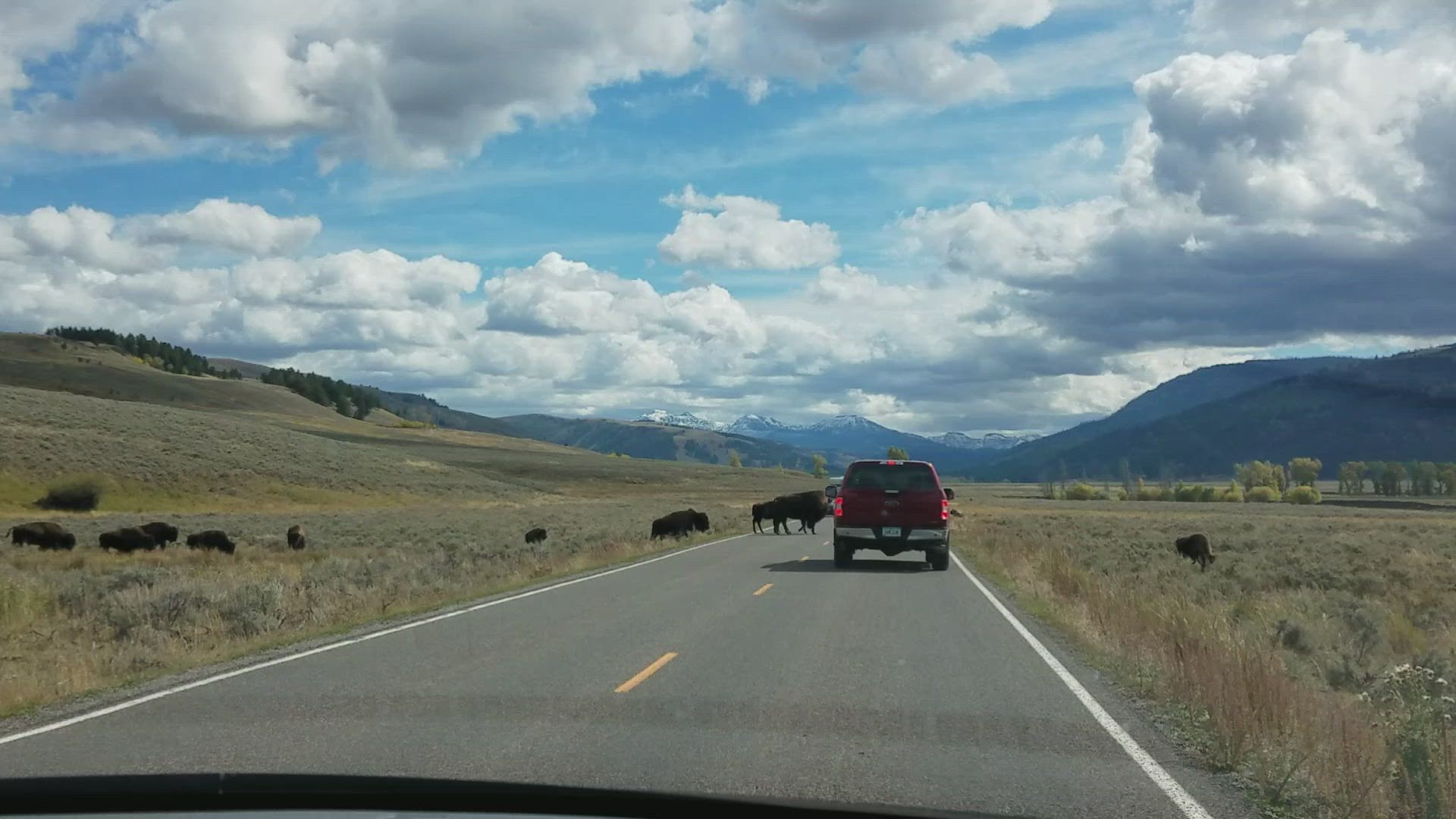A panoramic photograph captures a serene valley scene where a grey road with a yellow divider winds away into the horizon, bordered by lush green pastures. The road, more prominent in the foreground, is obstructed by a red four-wheel-drive vehicle, which appears to be navigating around a couple of bison standing nonchalantly on the pavement. Flanking the road, several bison graze, with six identifiable on the left side and another on the right. 

To the left, the landscape gently slopes into a hill adorned with scattered, dark green trees. On the far right, the terrain flattens out, presenting a lighter shade of green that contrasts the vibrant pastures. In the background, majestic mountains rise, capped with snow, under a sky that is partially overcast with a blend of dark grey and pristine white clouds, through which patches of blue sky peak. The entire scene conveys a tranquil coexistence between nature and human traversal, set against a backdrop of awe-inspiring natural beauty.